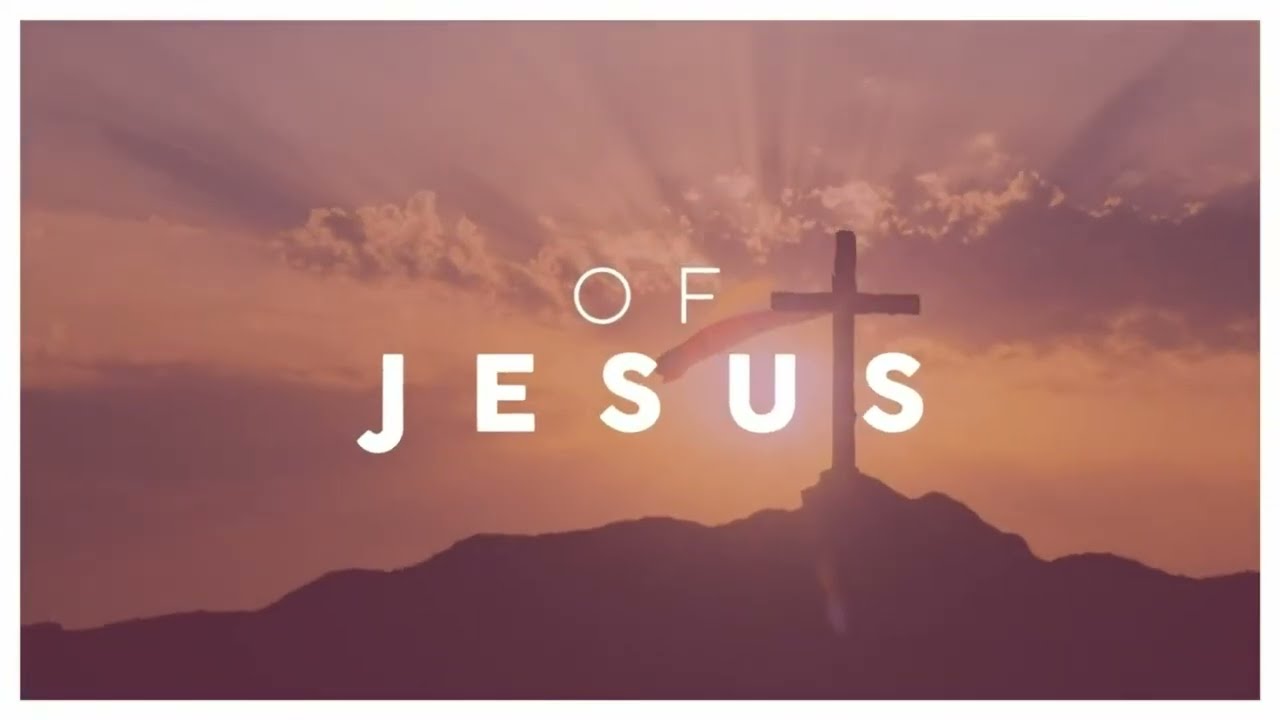The image is a horizontal, rectangular digital poster featuring a motivational outdoor scene. Dominating the composition is a mountain range or set of hills silhouetted against a sky that transitions from an orange and yellow dawn near the horizon to a purplish-violet hue higher up. Soft, puffy white clouds are dispersed across the sky, and rays of sunlight streak outward, suggesting a rising sun just out of sight. Positioned slightly to the right of center is a prominent, traditional cross with a draped garment fluttering towards the left. The entire image is overlaid with a light to medium brown filter, giving it a unified, warm tone. Centrally placed in bold white letters are the words "of Jesus," spread across two lines, with "of" appearing in a thin font and "Jesus" in a more robust style.